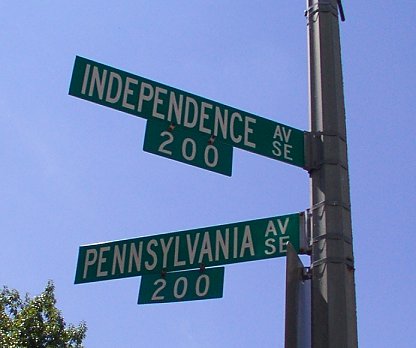This is a detailed photograph of a street sign taken during the daytime. A vertical metal post is oriented on the right-hand side of the image. The post holds two green street signs with white capital letters; the top sign reads "Independence Avenue SE 200" and the lower sign, positioned at a 90-degree angle, reads "Pennsylvania Avenue SE 200." The post is secured with cables that attach the signs firmly. In the background, a clear, sunny sky with a bluish hue can be seen, contrasting with the green foliage of a tree at the bottom left corner of the photo. The tree's leaves are lush and fully bloomed, indicating vibrant outdoor scenery. This setting suggests a location potentially in Washington, D.C.